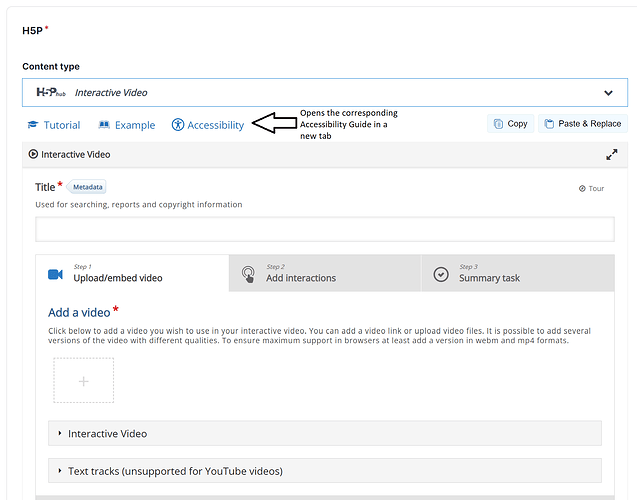This is a detailed caption for the provided image:

"The screenshot features the H5P Hub Interactive Video page, defined by a thin gray border on a white background. At the top, the words 'H5P Content Type H5P Hub Interactive Video Tutorial Example Accessibility' are prominently displayed. To the right of the term 'Accessibility,' a large black, outlined arrow points left, accompanied by text indicating it 'opens the corresponding accessibility guide in a new tab.' On the right-hand side, there are two buttons labeled 'Copy' and 'Paste and Replace' respectively. Horizontally across the screenshot, a gray bar displays 'Interactive Video' on the left. Beneath this bar, the section provides space for a title and includes options for 'Upload,' 'Embed Video,' 'Add Interactions,' 'Summary Tasks,' with additional buttons for 'Interactive Video' and 'Text Tracks Unsupported for YouTube Videos.'"